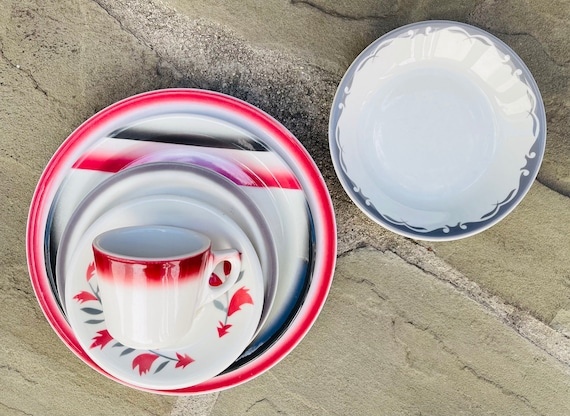The image displays a collection of intricately designed dinnerware set against a light brown, textured background reminiscent of sandstone or a natural surface. Centrally positioned to the bottom left is a large dinner plate with a prominent reddish-pink, black, and white striped border. Atop this large plate are two smaller stacked saucers, the uppermost featuring a detailed design of red flowers on a greenish vine. Perched atop is a white coffee mug, distinctively marked with a deep red trim around its rim. Towards the upper right side of the arrangement is a white bowl edged with a navy blue border adorned with delicate white swirls and dots, contributing to the artistic character of the scene.